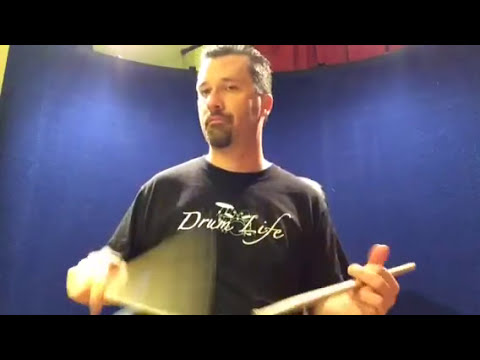This image features a white man in his late 30s to early 40s, playing the drums. The photograph is small and rectangular with thick black borders at the top and bottom. The man, centered within the frame, is slightly looking down at the camera, which appears to be positioned around his waist level. He has short salt-and-pepper hair and a brown goatee, accentuating his focused expression. His attire includes a short-sleeved, dark blue or black shirt emblazoned with the words "Drum Life" in white letters, along with an image of drums. In his hands, he holds a pair of drumsticks: one is clearly seen while the other is blurred in motion, suggesting active drumming. The indoor setting features a solid blue, curved backdrop and red curtains draped above it, indicating a studio or music room environment. The overall composition is vibrant with colors like black, blue, yellow, red, white, and tan adding depth to this dynamic scene of musical engagement.